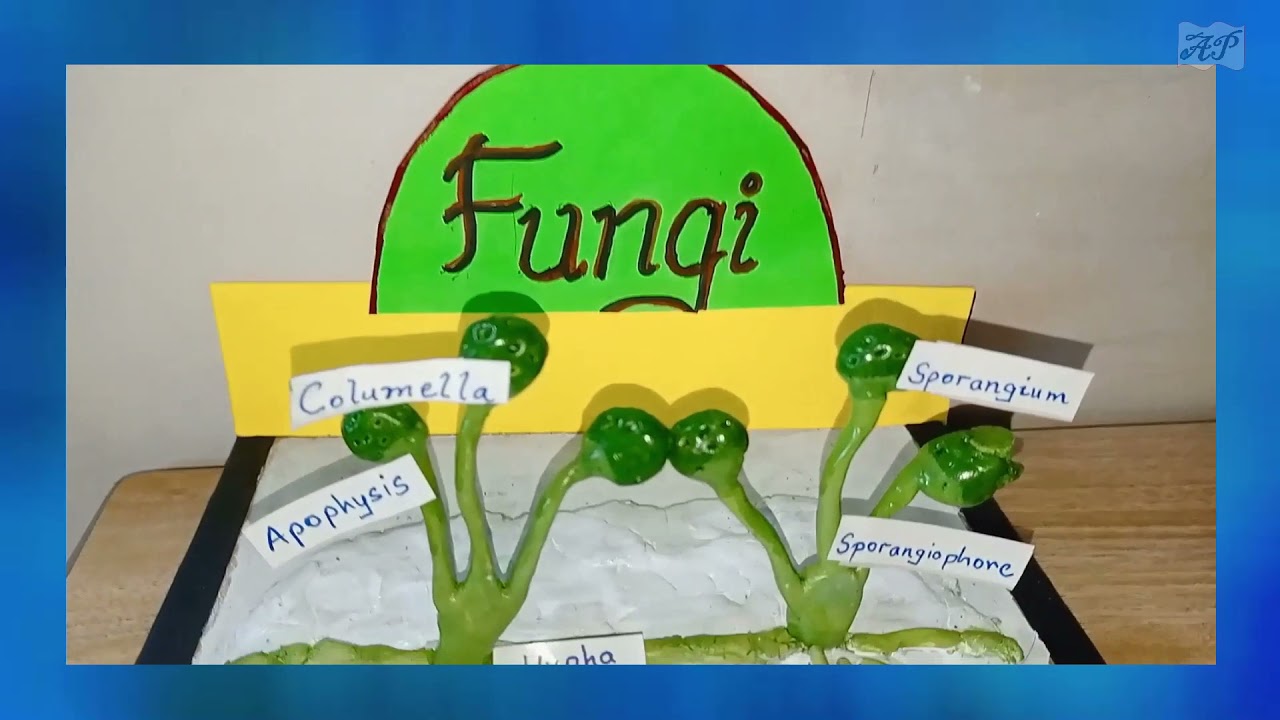The image depicts a detailed children's science project about fungi, set atop a wood table. The project, which appears to be made out of clay, features a small platform with green, plant-like structures emerging from it. Each structure is meticulously labeled with white rectangles containing blue text. From left to right, the labels read "Apophysis," "Columella," and another label partially visible ending in "HA." Additional labels to the right identify parts as "Sporangium" and "Sporangiophore." A yellow rectangular piece of poster paper stands behind these plant structures, with a green, arched poster paper above it that bears the word "Fungi" written in black marker. Notably, in the upper right corner of the display, the initials "AP" are visible in cursive within a blue, rectangular design. The background features a plain white wall, further emphasizing the colorful, educational display.